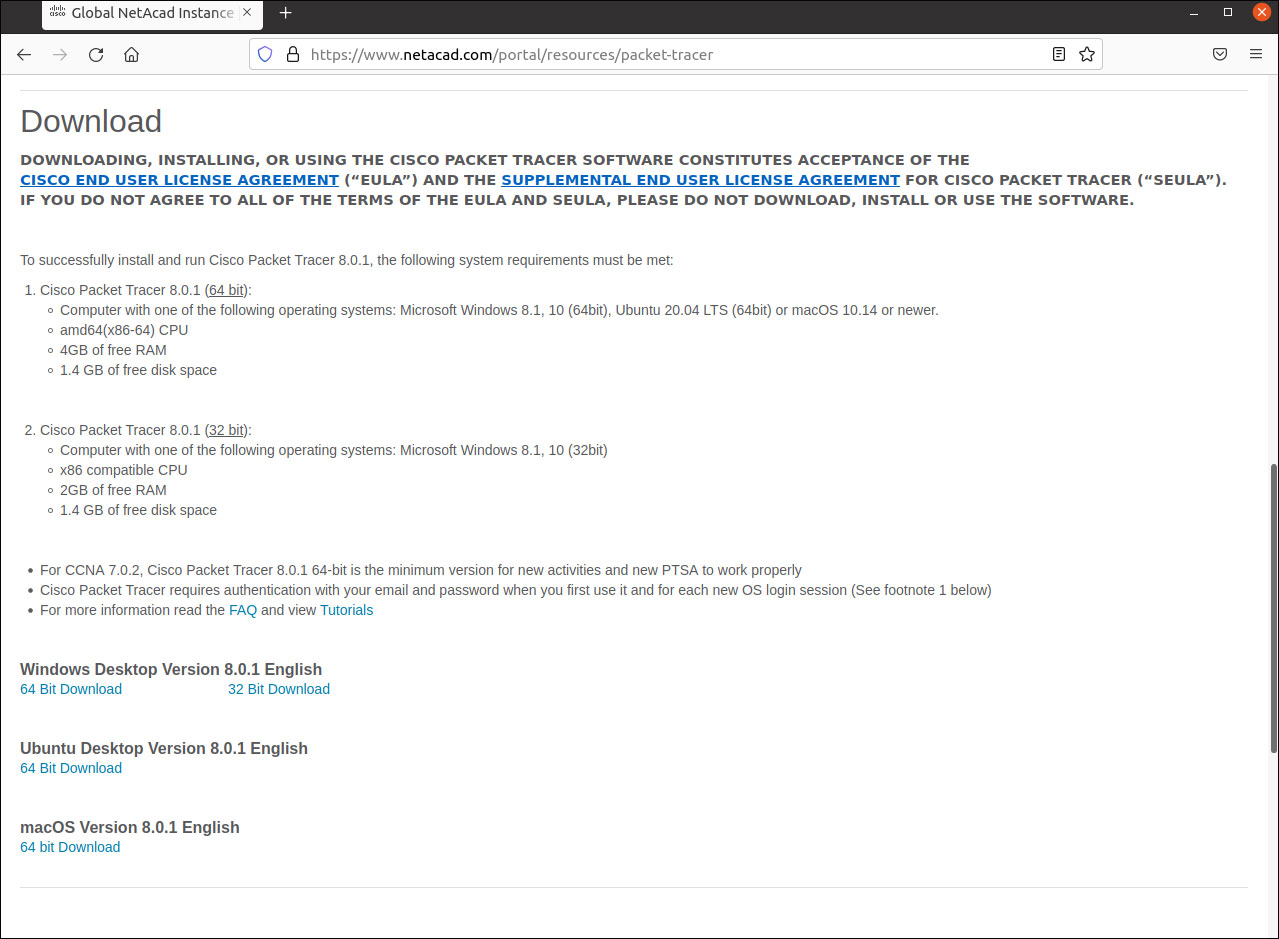Screenshot of a web page section displaying a user interface and document details. In the top left corner, a white box labeled "Global NetCAD Instance" is partially cut off, with an "X" icon beside it for closing the box. Below this is the browser search bar, centered and showing the URL: netcad.com/portals/resources/packet-tracer. To the left of the search bar, there are navigation buttons for home, refresh, and back & forward functionalities.

The main body of the web page displays a downloadable document. At the top of this section, the word "Download" is prominently written in black. Below this header, a disclaimer is presented, featuring two hyperlinks: one for a "Supplemental End User License Agreement" and another for the "Cisco End User License Agreement." Further down, the page provides instructions on accessing the web page and outlines the computer requirements needed for the associated application.